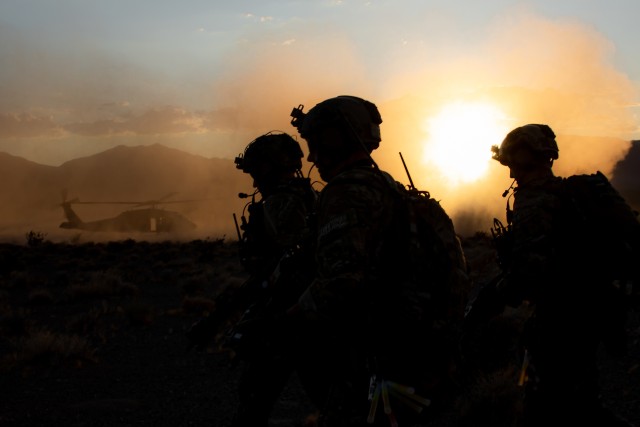In this evocative photograph captured at sunset, three silhouetted soldiers, distinguished by their helmets and attached microphones, stand prominently in the foreground. The two soldiers in front are side by side, while a third soldier is positioned slightly behind them. Their dark figures are backlit by the setting sun, rendering their detailed features indistinguishable but casting a dramatic and somber tone over the scene. Each soldier is equipped with headsets and other gear, indicating active communication with their team. In the background, a helicopter rests on the ground, partially obscured by swirling dust and smoke, likely suggesting a recent landing. The serene mountain range and a few light clouds frame the scene, contrasting with the rugged and intense atmosphere created by the soldiers and the helicopter.